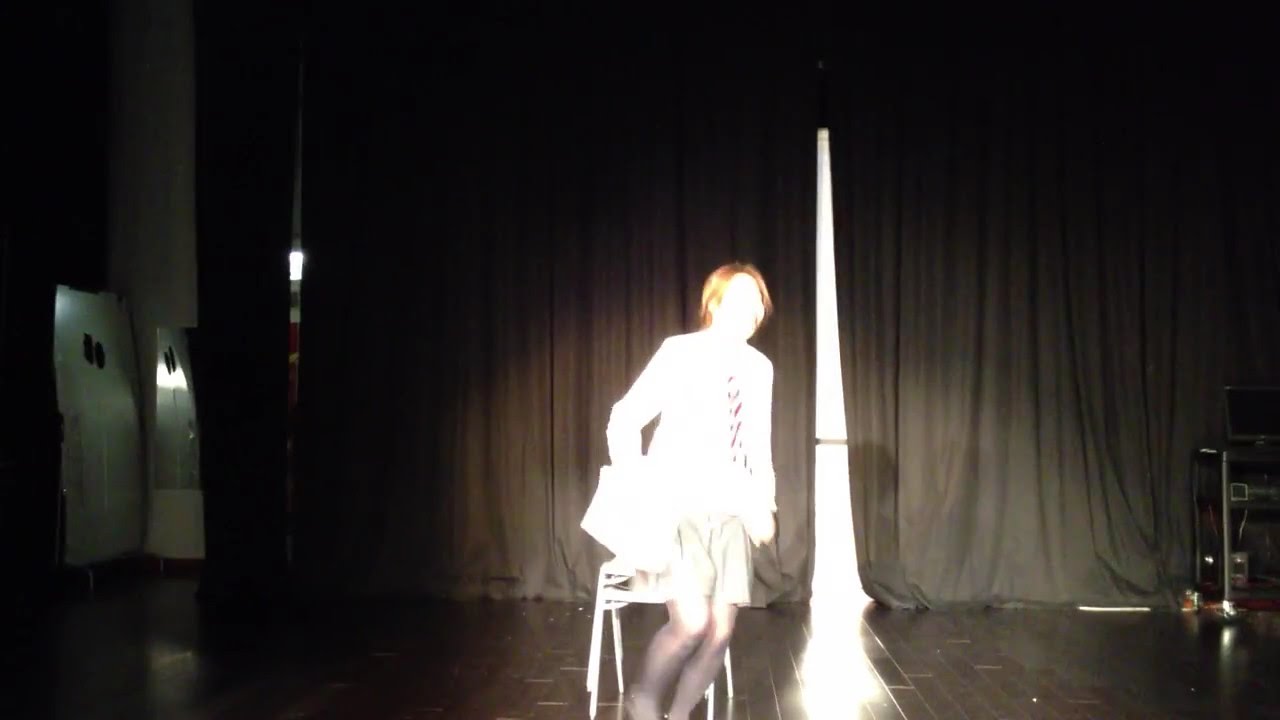The image captures a young lady with red hair, wearing a white skirt and stockings, standing on a theater stage. She appears to be involved in some kind of performance or practice, but the exact nature is unclear. The background features a slightly opened theater curtain with a visible gap extending towards the floor. The lighting is extremely bright, obscuring her face and making it difficult to see any facial features, thus rendering her age indeterminable. She seems to be walking away from a chair, possibly moving to another part of the stage or towards the audience. On the right side, there's a cart that may be holding a computer or other technical equipment, while on the left, an open door extends onto the stage. The overall scene is dominated by an overwhelming brightness that washes out finer details and makes certain elements, like what she is holding, indistinguishable.